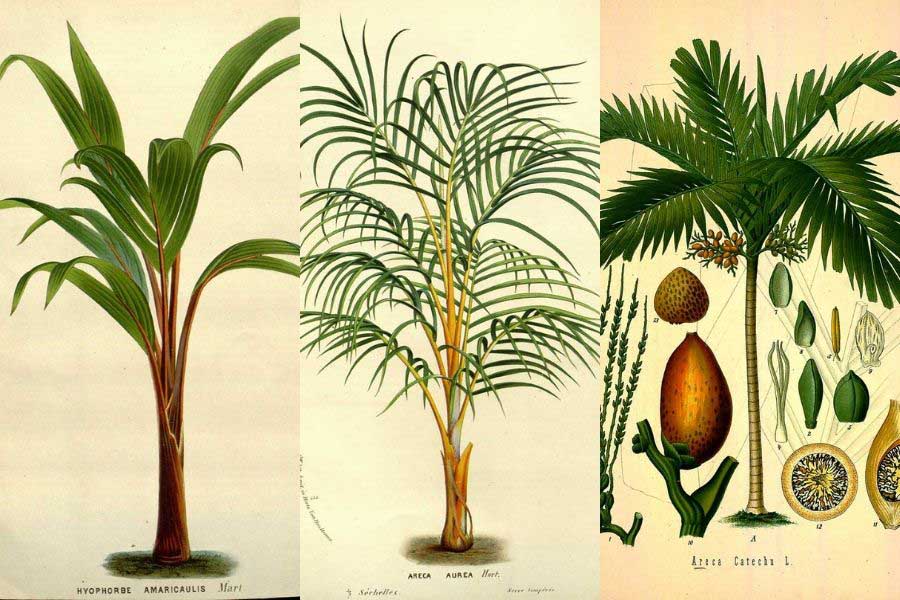This image is a triptych of vintage botanical illustrations, each panel depicting a different species of palm tree. The leftmost illustration features a palm tree with a robust brown stalk and darker leaves, labeled "Hiaforte Americaulis - Mary." The middle panel showcases another palm tree with a yellowish-orange stalk and more delicate, spindly fronds, identified as "America Aria." The rightmost drawing is the most detailed, depicting a palm tree along with various anatomical details such as seeds, cutaways of seeds, and buds, under the label "Africa Catera." These highly detailed illustrations, reminiscent of classical scientific drawings, would likely be found in an old horticulture book, illustrating different palm species and their unique characteristics for educational purposes.